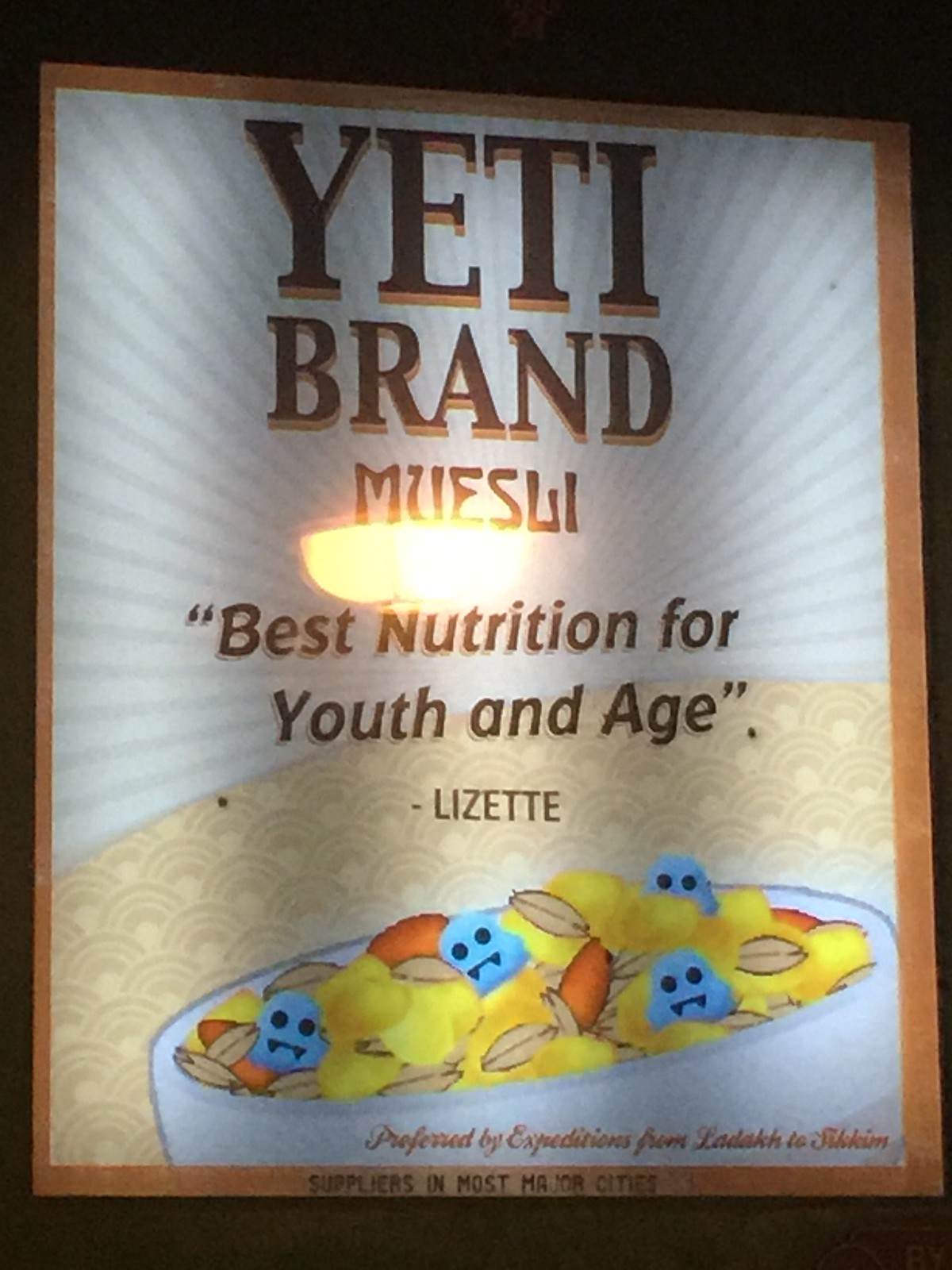The image depicts the cover of a cookbook titled "Yeti Brand." The title is prominently displayed at the top in bold black letters, outlined in a brownish hue. Just below the title, the word "MUESLI" is featured in a uniquely styled font, catching the viewer’s eye. 

Underneath the word "MUESLI," there is a reflection of a yellow light, highlighting the area. Following this is a quotation, "Best Nutrition for Youth and Age," attributed to "Lizette." This quote is also prominently displayed in a readable font.

The background of the cover is artistically designed with a blend of gray hues. At the top, gray horizontal lines are intersected by vertical lines, creating a dynamic pattern. Moving downward, the background transitions into a series of tan circular shapes. 

The focal point of the cover is a bowl in the center, filled with a mix of yellow, blue, and orangish-brown contents, encased in a brown outer cover. The bowl and its contents are set against a stark black background, adding contrast and drawing attention to the vibrant colors within the bowl.